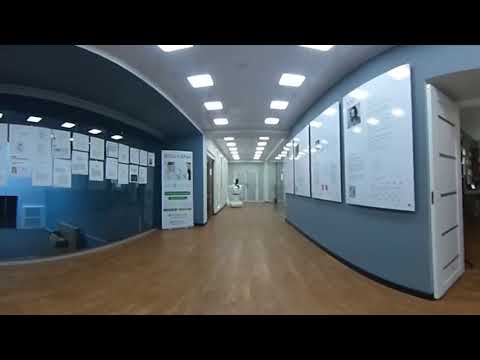The image depicts an office setting, possibly medical, with a black border at the top and bottom. The medium brown wood floor or laminate extends throughout the space. On the left side, there's a glass wall adorned with about 12 to 15 white papers and notices taped up. Behind this glass wall, there's a small ventilation unit. Continuing into the hallway, the ceiling features rows of fluorescent lights, approximately 14 to 16 in total, guiding the eye down the corridor. On the right side, a blue wall showcases several large informational plaques or posters, with some describing human figures accompanied by paragraphs of text. Adjacent to this blue wall is an open white doorway leading into another room, which remains out of view. At the end of the visible part of the hallway on the left side, there's a door that is hard to make out due to its distance. The atmosphere is lit evenly with detailed elements that suggest this is a functional office, complete with various informational displays and practical lighting.